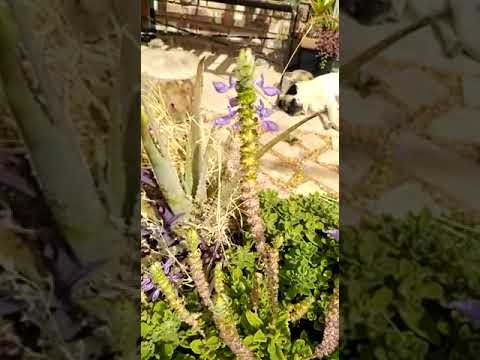This outdoor image captures a chaotic yet intriguing assortment of plants. Dominating the scene is a bushy plant about a foot tall, composed of various stalks adorned with small leaves. These leaves are greener at the top and transition to a whitish hue towards the bottom. The plants appear to be rooted in a pot and share space with an aloe vera plant, distinguishable by its sharp tendrils and some surrounding purple leaves. Also present are vertical stalks studded with buds, resembling fuzzy poles, adding to the diverse vegetation. The backdrop includes a bench, hay-colored areas, a metal fence, and some stepping stones partly overtaken by grass, suggesting a mix of a patio and farm-like setting. The predominant colors are green and yellowish, with a distinct vertical focus, possibly hinting at the image being taken with a phone. The image also features a grayed border that elongates and frames the central chaotic plant scene.